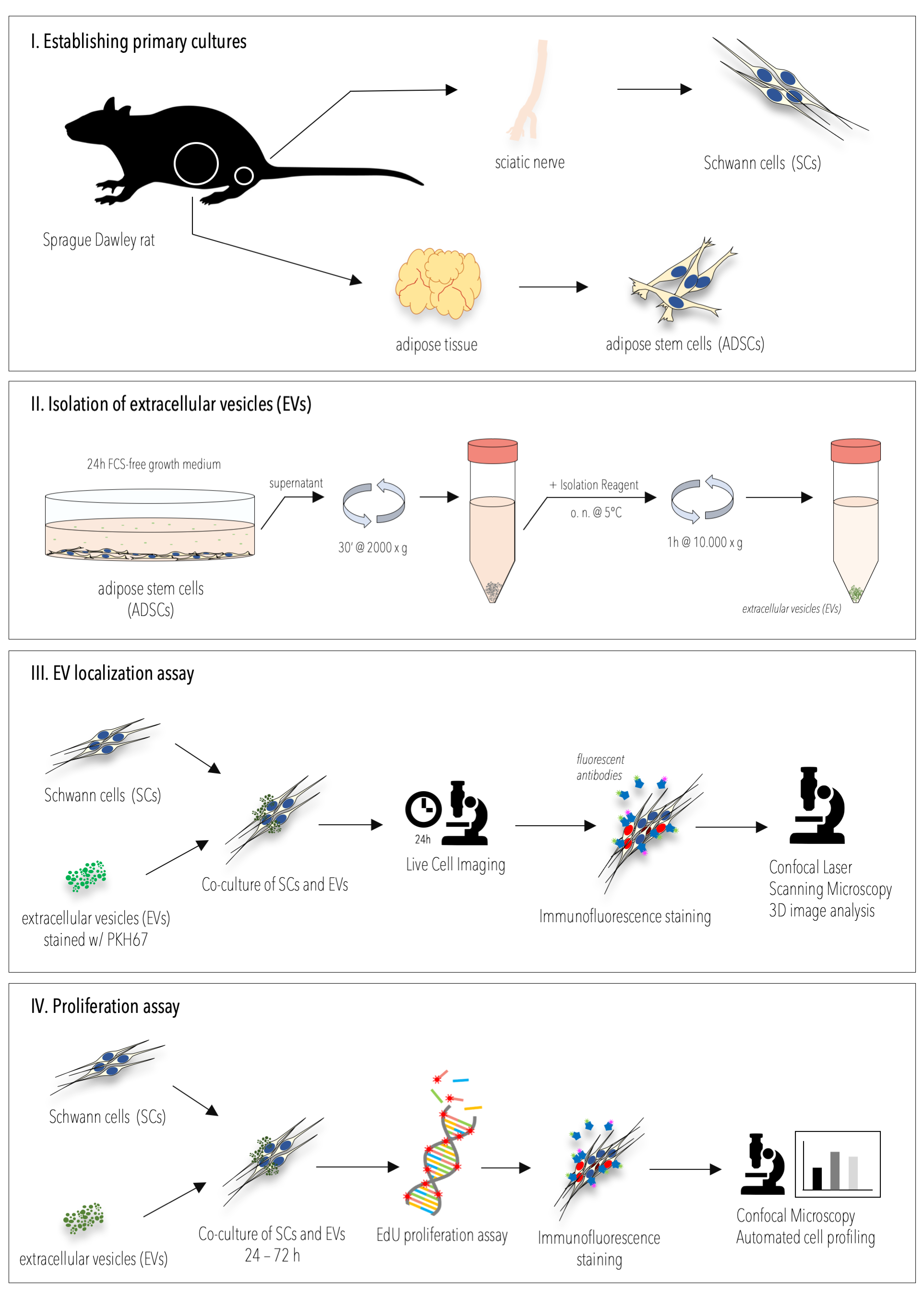The image is a detailed chart illustrating the steps of a scientific process utilizing Sprague-Dawley rats. The first step, labeled "1. Establishing Primary Cultures," features a silhouette of a rat with circles over its sciatic nerve and adipose tissue, indicating the source of the samples. Arrows point from these circles to Schwann cells derived from the sciatic nerve and adipose stem cells from the adipose tissue. 

The second step, "2. Isolation of Extracellular Vesicles (EVs)," shows a Petri dish containing stem cells, accompanied by arrows moving towards vials with pink liquid, indicating the separation and collection process of EVs.

In the third step, "3. EV Localization Assay," the chart details the co-culture of Schwann cells (SCs) with EVs. This step includes intricate illustrations of live cell imaging, immunofluorescence staining, and laser scanning microscopy for 3D image analysis, demonstrating the localization of EVs within the cells.

The fourth and final step, "4. Proliferation Assay," depicts various stages leading up to confocal microscopic automated cell profiling. This includes images of Schwann cells, extracellular vesicles, and other technical illustrations, culminating in a sophisticated analysis of cell proliferation.

Throughout, the chart utilizes visual aids such as microscopes, cells, and scientific annotations to represent each phase of the process in a highly detailed and structured manner.